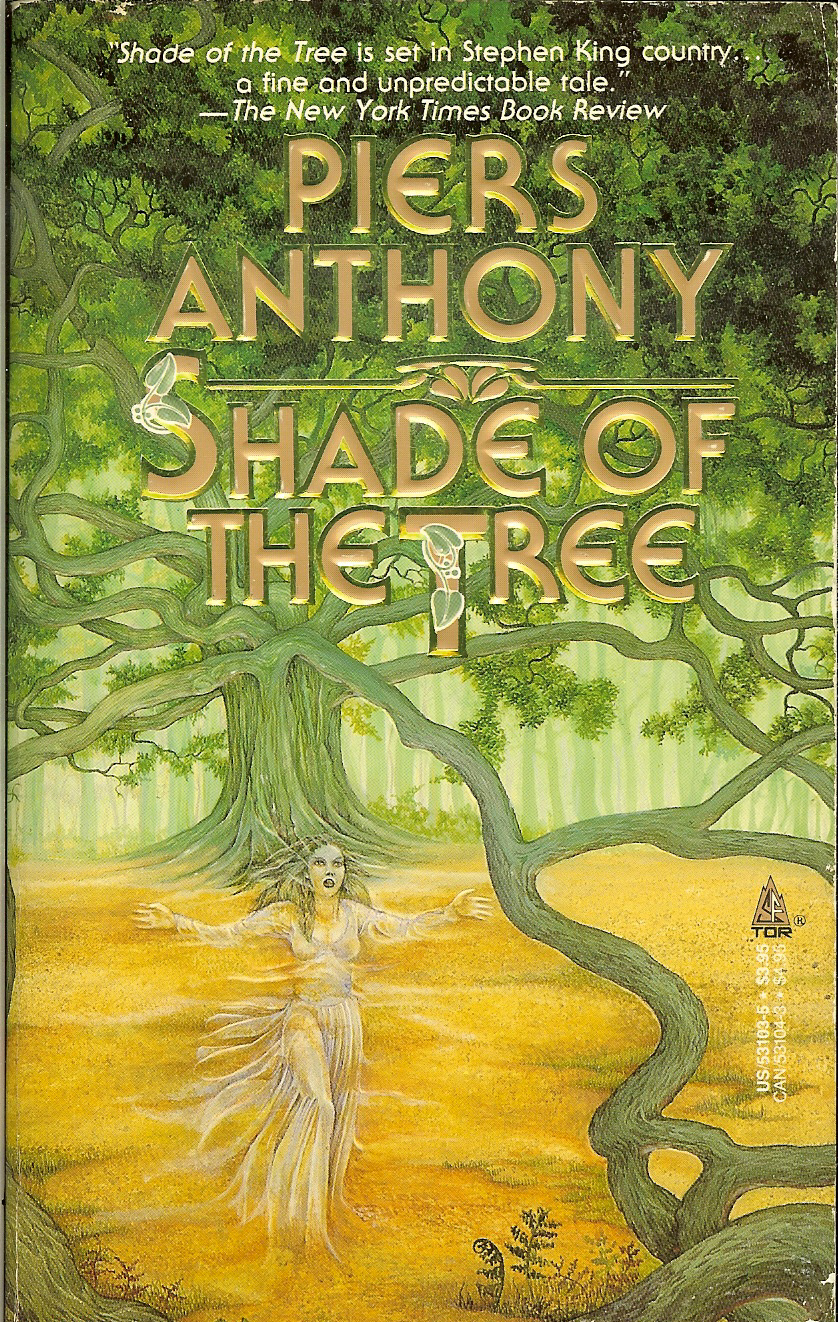The cover of the book, primarily hand-drawn with detailed artwork, prominently features a large tree with sprawling, intricate branches extending across the front, shaded in multiple greens to represent the leaves. At the bottom, a spectral, ethereal woman in a flowing white dress reaches outwards, set against a yellow field. The title "Shade of the Tree" and the author's name, "Piers Anthony," are embossed in gold, raised lettering. At the top, there is a printed endorsement from the New York Times Book Review in white text, stating: "Shade of the Tree is set in Stephen King country, a fine and unpredictable tale." Additionally, sales information is provided on the right side in white text, indicating the US price ($3.95) and Canadian price ($4.95).